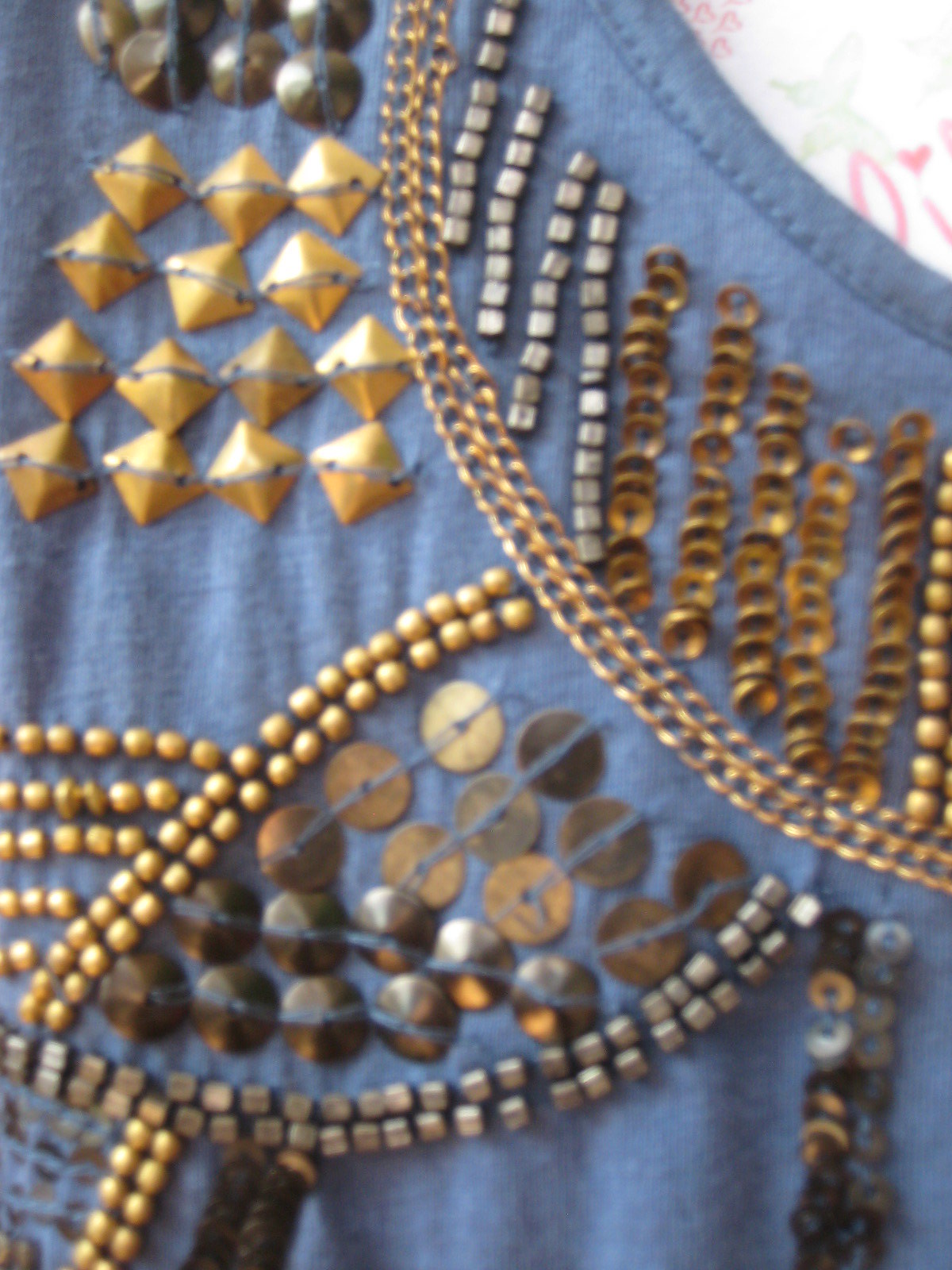This photo showcases a blue fabric, most likely a shirt, lying on paper adorned with heart designs. The shirt is intricately decorated with a variety of beads, jewelry, and metallic embellishments. At the top right, we can see the neck hole of the shirt, indicating its orientation. Starting from the upper left, there are bead-like chimes sewn into the fabric. Below these, rows of diamond-shaped or cube-like beads span the shirt, each bead artfully sewn at specific angles to create a shimmering, 'diamond' effect. Adjacent to these are multiple chains, approximately ten, draping down the fabric. Surrounding the chains are numerous small gray metal pieces, possibly symbolic shapes or rings, meticulously sewn into the fabric. The detailed arrangement includes additional metallic beads and sequins, all contributing to an ornate and intricately decorated garment. The overall composition shows the shirt slightly turned sideways, highlighting the detailed craftsmanship in each attached piece.